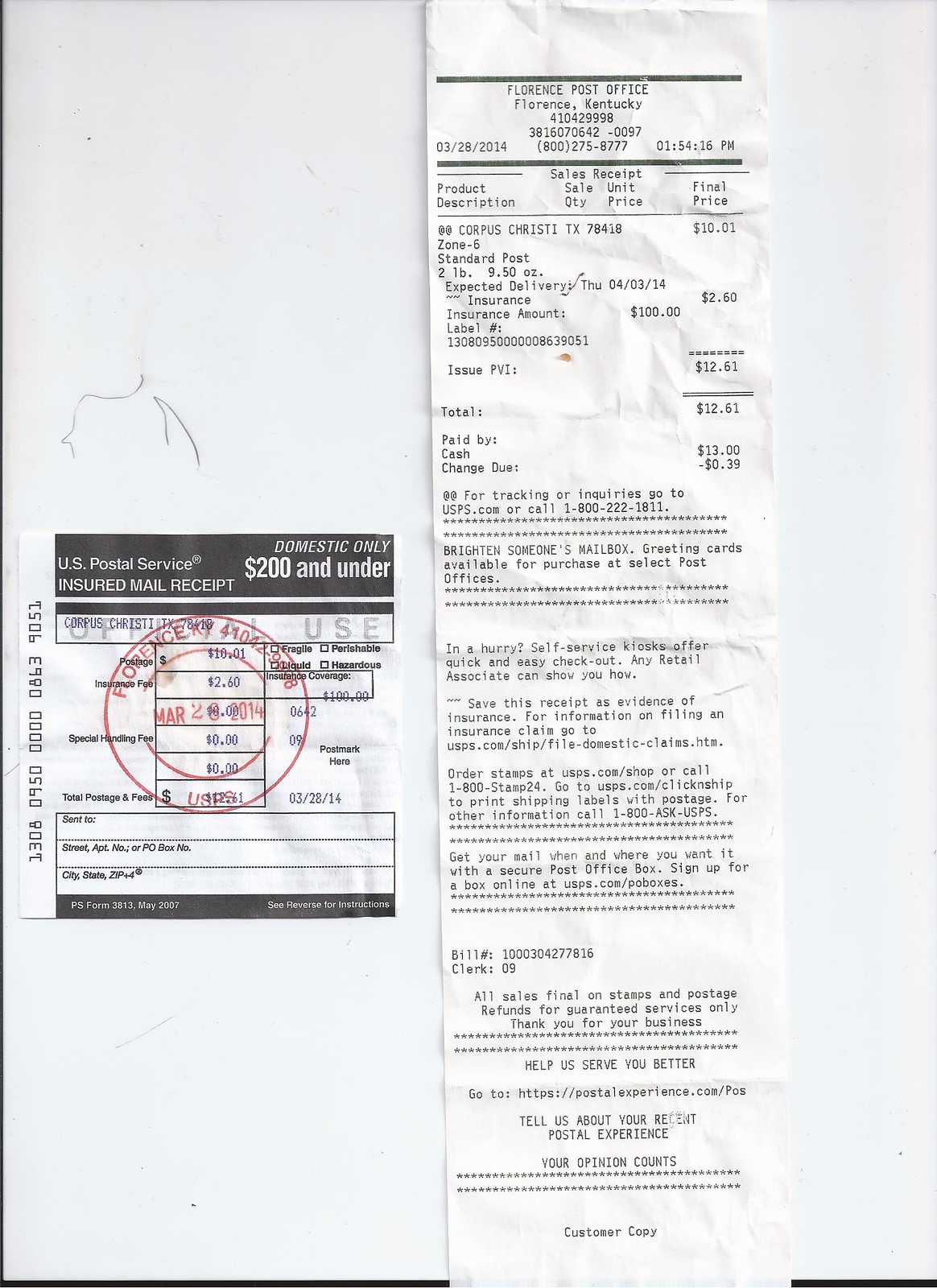This is a detailed color photograph showcasing two United States Postal Service documents on a white desk background. Dominating the right side of the image is a long, vertically arranged receipt from the Florence Post Office in Florence, Kentucky. This receipt features comprehensive details, including the shipment from Corpus Christi, Zone 6, costing $10 with an additional $2.60, totaling $13, paid in cash. The receipt, dated March 2, 2014, also includes standard policies and postage information towards the bottom. Positioned centrally on the left side of the image is a smaller, square, insured mail receipt with a striking red circular stamp indicating domestic only insurance coverage up to $100. This receipt also contains areas for addressing, although these fields remain blank. Both documents offer a clear depiction of postal transaction details and confirm the insured and paid postage from this specific mailing instance.